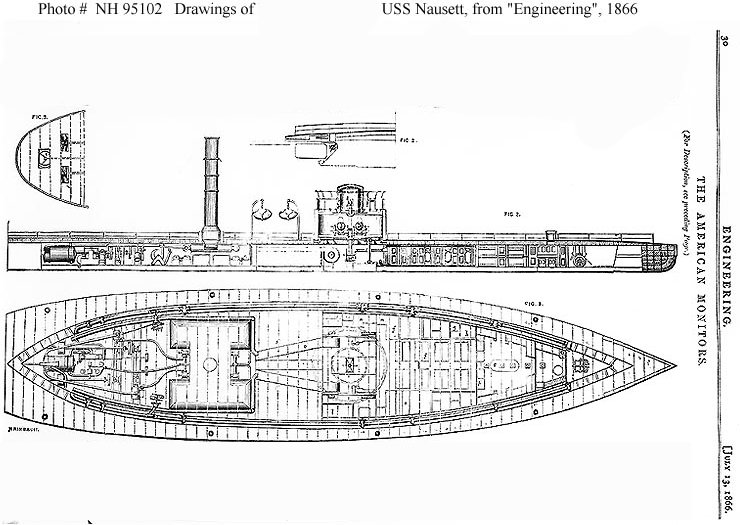This detailed, black-and-white engineered drawing from July 13, 1866, titled "The American Monitors," features the naval warship USS Nauset. The image, identified by photo number NH-95-102, presents both a top view and a side view of the ship. The top view reveals the deck configuration, squared at the rear and tapering to a point at the bow, with various cabins and compartments likely designated for storage and operational functions, including potential weapon storages like black powder and boiler water reserves. The side view provides insight into the ship's structure, showcasing a prominent smokestack indicative of its steam-powered boiler system. The drawing meticulously illustrates the different areas within the vessel, likely including quarters for soldiers and essential power units. Notably, the image emphasizes the sophisticated engineering of the era, capturing the intricate details of the warship's design and functionality.